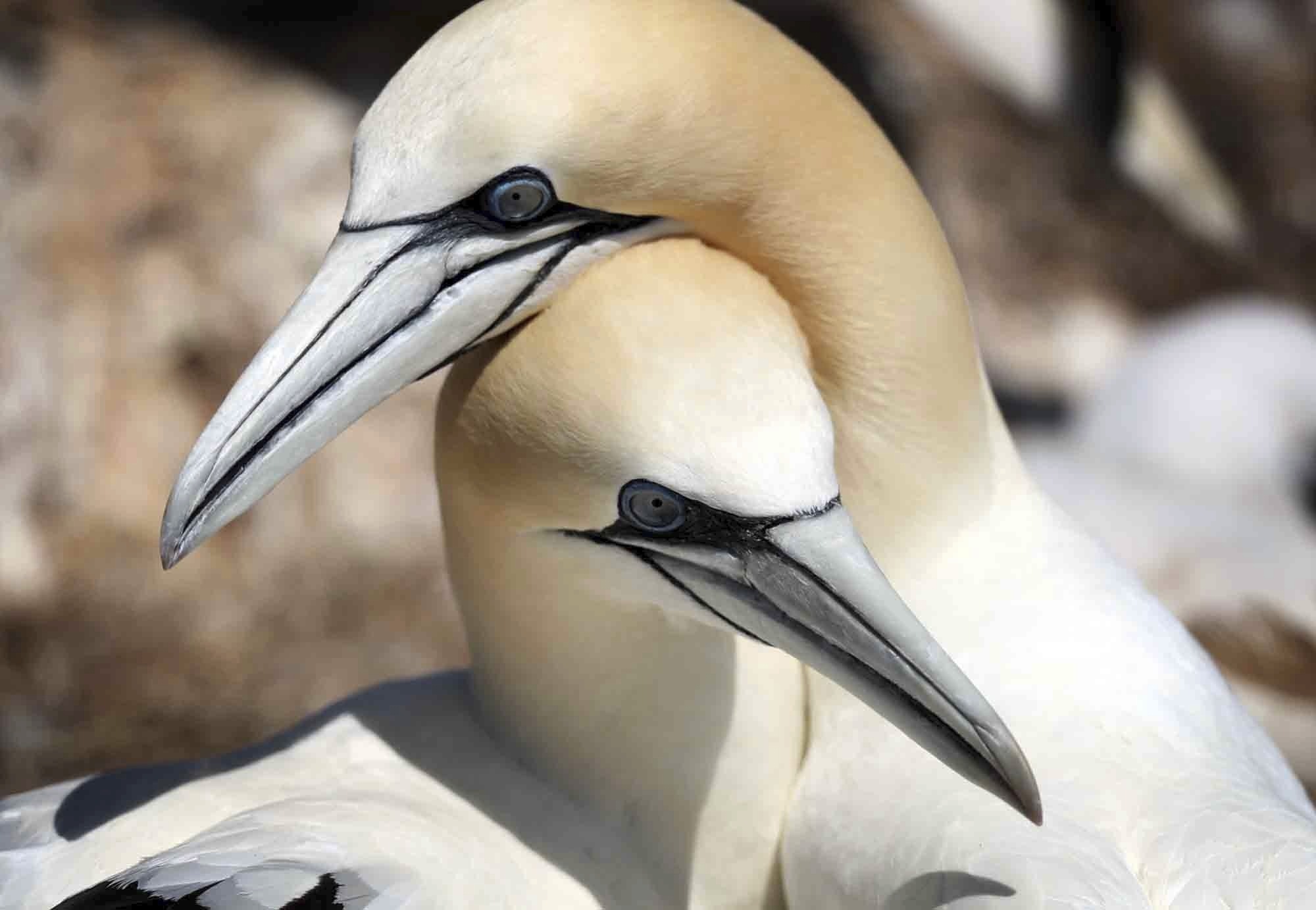This close-up, color photograph, set in landscape orientation, depicts an intimate moment between two birds, seemingly embracing. Both birds belong to the same species, featuring predominantly white feathers contrasted by subtle cream or beige tones on their heads and necks. The birds also have black mask-like markings around their eyes and on their long, pointed white beaks, with some black lines running down the length of their beaks. The bird positioned on top appears larger, with its head facing left and its neck gracefully wrapped around the other bird’s head. The bottom bird is tucked under the top bird’s neck, facing right, with part of its back visible on the left side of the image. The setting hints at a rocky, coastal environment, as evidenced by the blurred background interspersed with brown, black, and white objects. The photograph appears to be taken around midday to early evening, illuminated by the soft shadows cast on the birds. The candid composition captures not only the physical features but also the tender interaction between the avian pair.